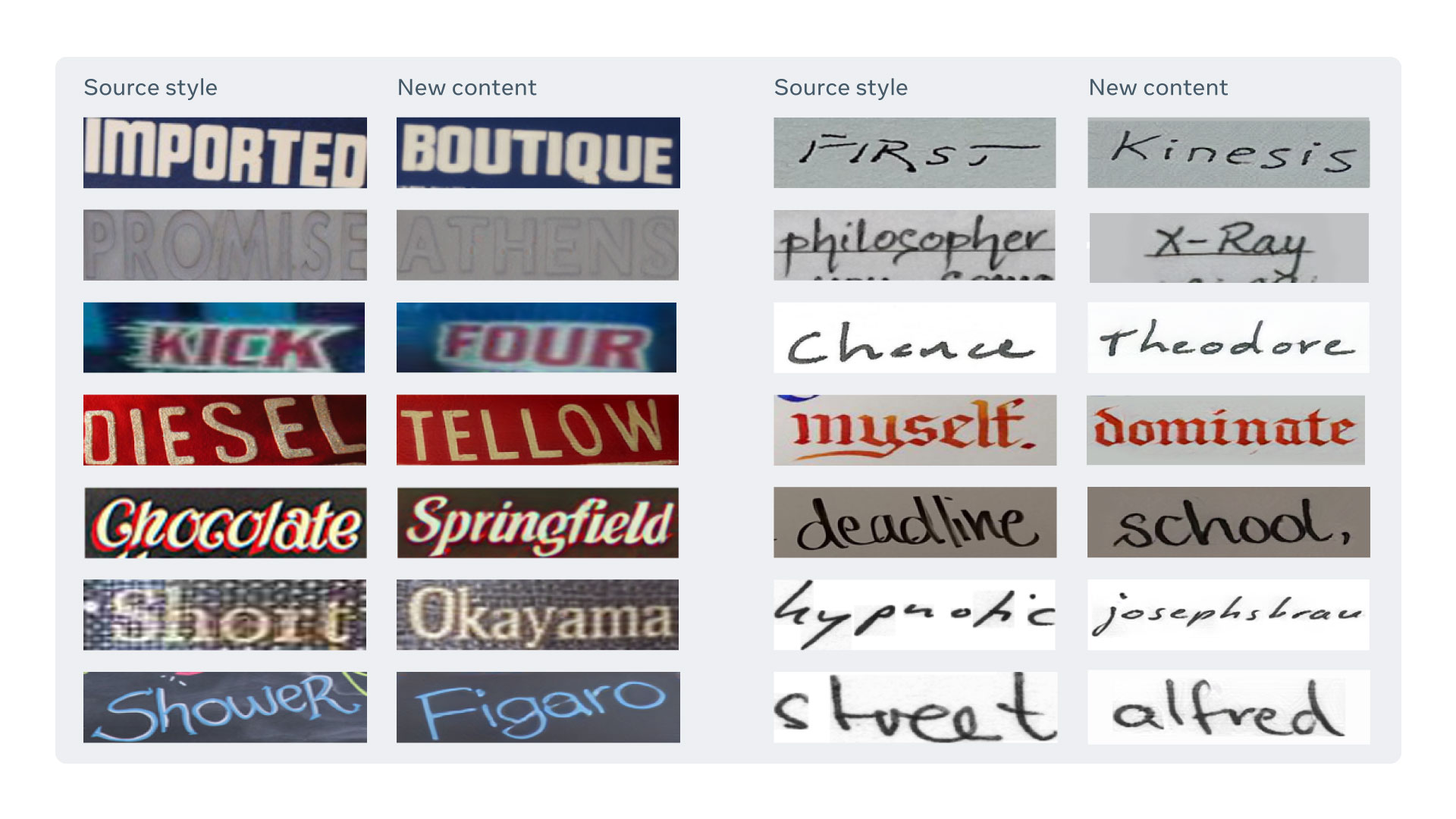The image is a detailed collage comprising various CAPTCHA words, designed to verify that the user is not a bot. The collage is organized into a grid with four columns and seven rows, each containing rectangular images of words printed on documents. Overall, the collage is rectangular, with the longer sides at the top and bottom, and a light gray background and borders.

In the first row, starting from the top left and moving to the right, the words are IMPORTED, BOUTIQUE, FIRST, and KINESIS. The second row features PROMISE, ATHENS, PHILOSOPHER, and X-RAY. The third row displays KICK, FOR, CHANCE, and THEODORE. The fourth row includes DIESEL, TELLO, MYSELF, and DOMINATE. The fifth row offers CHOCOLATE, SPRINGFIELD, DEADLINE, and SCHOOL. The sixth row lists SHORT, OKAYAMA, HYPNOTIC, and JOSEPH, SPROUT. The final, seventh row reads SHOWER, VIGORO, STREET, and ALFRED.

Each word is encased in a banner-like rectangular photo, maintaining the collage's uniform structure and seamlessly blending into the light gray backdrop.